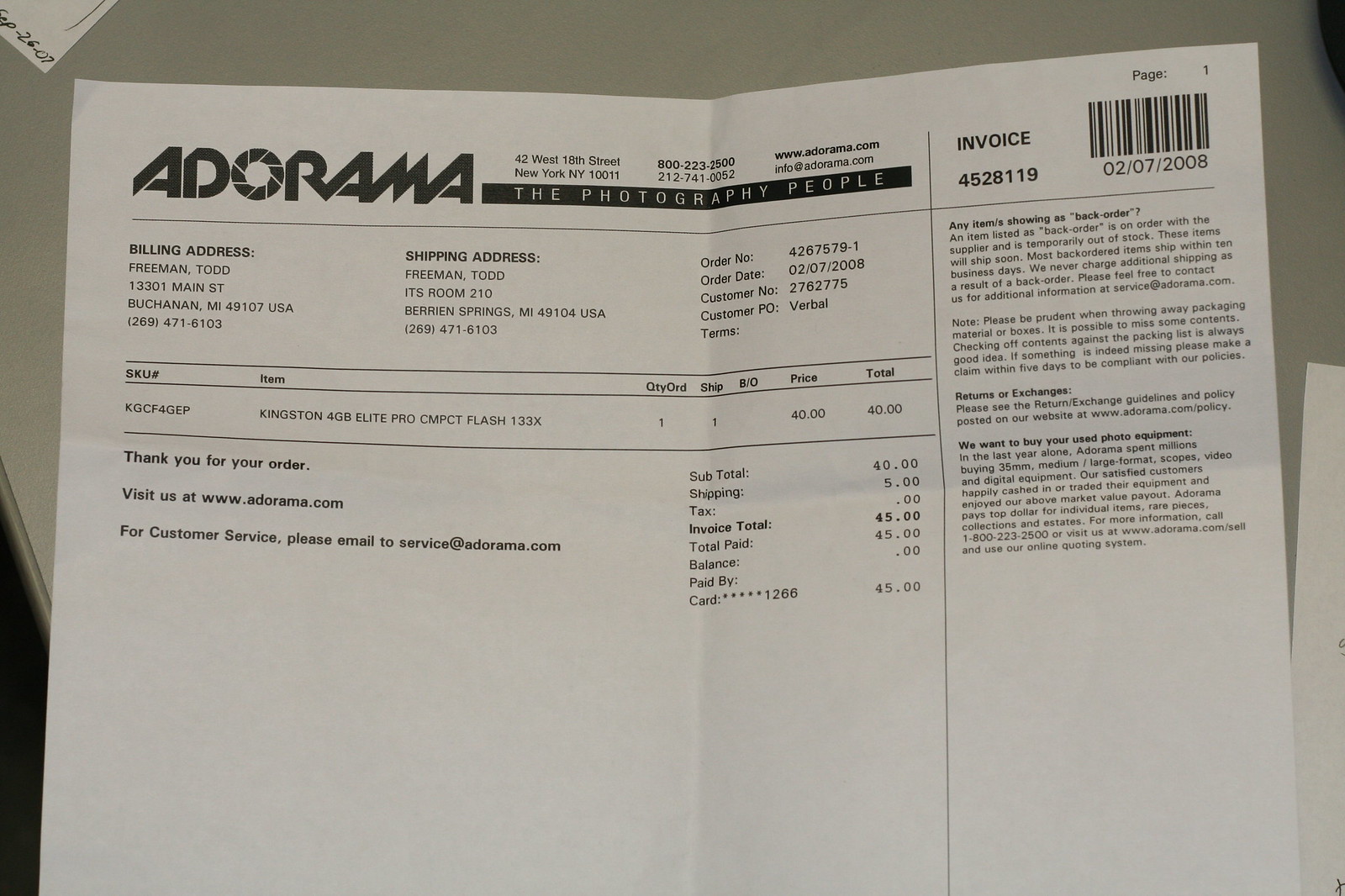This is a color photograph of a gray desktop featuring a rectangular piece of paper centered on it. The paper is an invoice from Adorama, the photography company, printed on white with black lettering. At the top, it prominently displays "Adorama, The Photography People" followed by the label "Invoice" and a barcode. Below this, various details are meticulously listed: the billing and shipping addresses, the order number, the date, the customer number, and the customer PO terms. Additionally, the document enumerates the items ordered along with their SKU numbers, prices, and a total amount of $45. A paragraph beneath the listed items outlines the terms and conditions. To the right edge of the image, a second piece of paper is partially visible, hinting at more documentation. The invoice also includes a note of appreciation, inviting customers to visit www.adorama.com and providing an email for customer service inquiries: service@adorama.com.